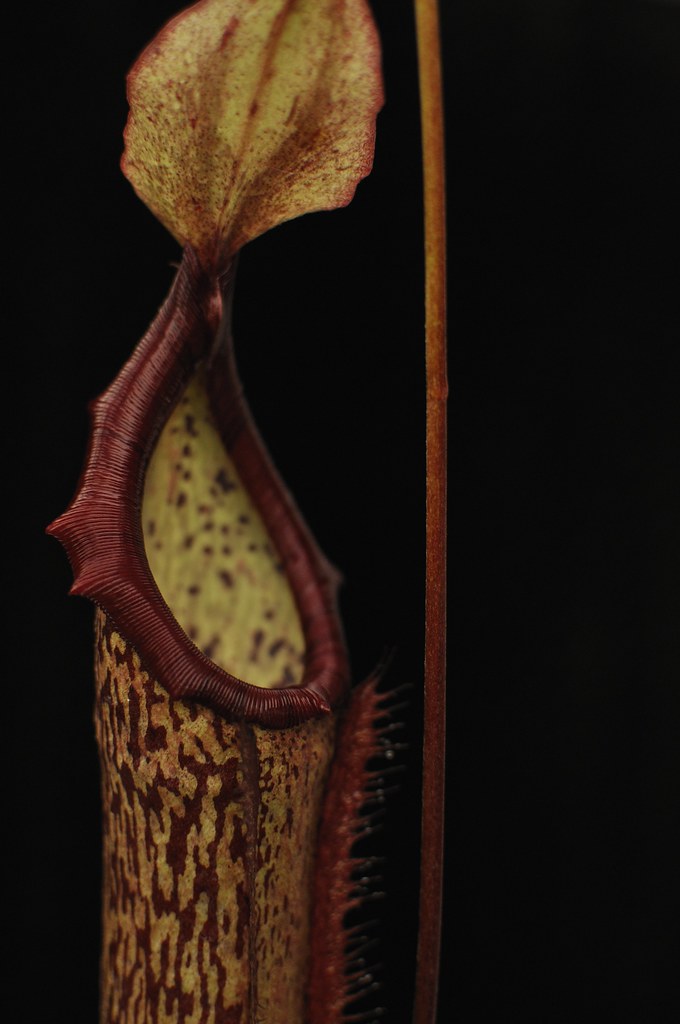In this detailed side-view photograph, we observe a fascinating bell-shaped flower, likely a carnivorous plant designed to trap insects. The apex of the flower features an open flap that resembles a small cover, revealing a lighter-colored interior adorned with vertical grainy lines and tiny black dots. These details suggest the plant's interior is structured to ensnare prey. 

The exterior of the flower displays prominent, vertically splashed black lines that contrast against its overall coloration. Along the bottom right side of the flower, small, spike-like protrusions are visible, adding to the intricate texture of the plant. To the right of the flower, a tall, vertical stem ascends from the center, yet it seems detached from any visible foliage, creating a striking visual element in the composition.

Most notably, the flower's outer rim is accentuated by a vibrant, ruby-red lip-like structure, enhancing its captivating appearance. Overall, the image centers on this intriguing bell-shaped plant, highlighting its unique adaptations for capturing insects.